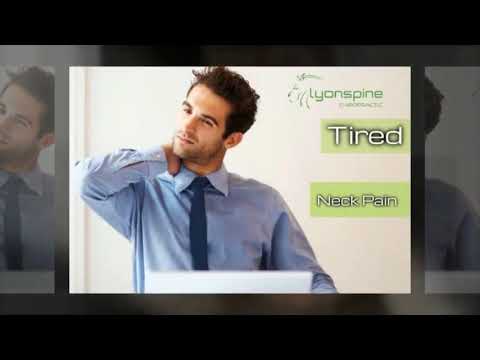The image is a horizontally oriented, low-quality color photograph inset against a larger replica of the same photograph with a darker overlay. It features a man wearing a blue button-down shirt and a dark blue tie, sitting at a workstation. He has dark, longish hair and a black beard. His right arm is bent so that his hand is cradling his neck from behind, giving the impression that he is experiencing neck pain. Surrounding the central image, there are darkened areas on the top and bottom and lighter areas on the sides.

On the right side of the main image, prominently displayed, is a large green rectangle with the word "tired" in white text with a black outline. Below that, another green rectangle contains the partially obscured words "neck pain" in similar typography. In the top right corner, there is a logo in green text that reads "Lion's Spine" with a swirly vertebrae design to the left of the text. The overall composition and repetitive background emphasize the man's discomfort, making it clear that the image advertises relief for neck pain.